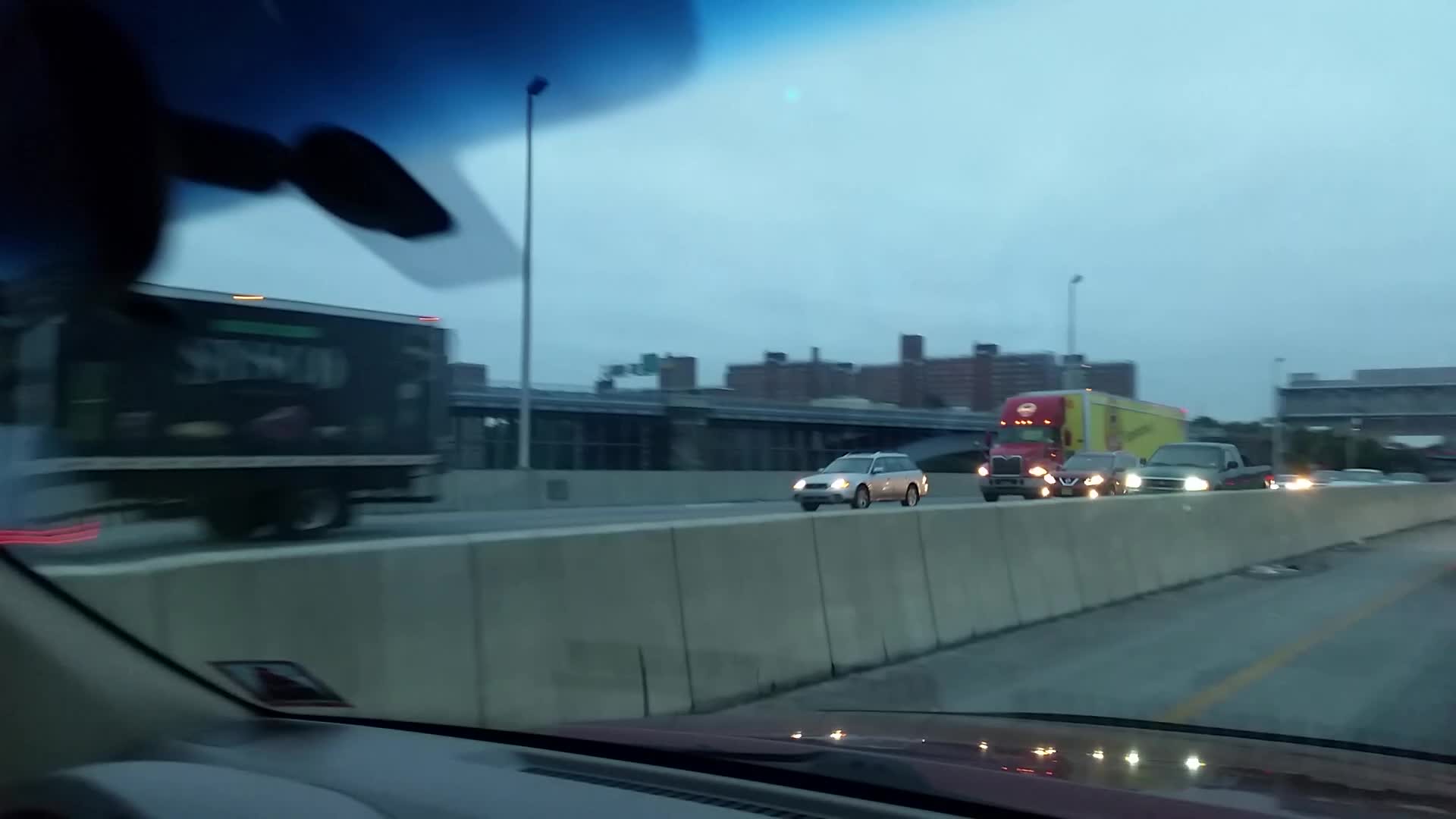In the image, a girl appears prominently in the foreground, possibly taken from the interior of a car. The photo was captured through the front windshield, showing a busy roadway. The road depicted seems to be a four-way intersection with various cars traveling in the opposite direction of the photographer. Notably, a red and yellow track is visible alongside the road. Additionally, buildings line the sides of the street, and there are street lamps present, though they are unlit.